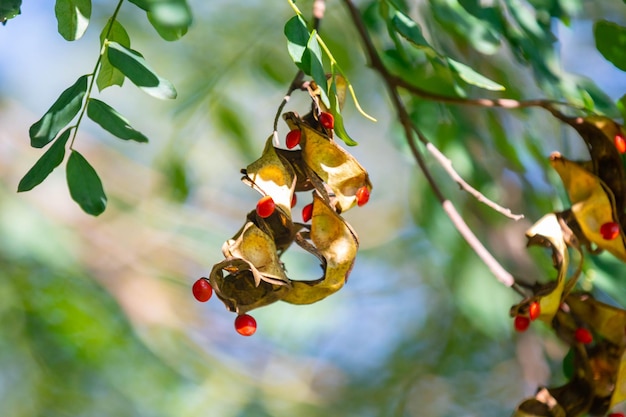The image is a close-up of a branch from a tree or plant, with a central focus on leaves and small berries. The scene is rectangular and wider than it is tall. On the left side, small green leaves hang down from the stem. In the center, there are yellowish-brown, dried-up leaves interspersed with small, red, rounded berries that resemble cranberries but are flatter. These berries appear to be on the verge of rotting. Additional branches with green leaves and more of these distinct red berries extend towards the right side, where the image fades slightly. The background features a blurred mix of blue and green tones, suggesting more trees or the sky, with some light rays filtering through. This out-of-focus backdrop provides a soft contrast to the detailed, albeit distressed, foreground foliage and berries.